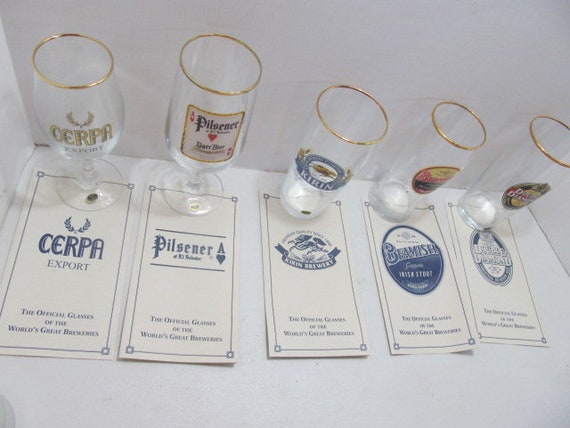This detailed photograph captures an organized beer tasting contest setup. Five clear glasses, each adorned with a gold rim, stand vertically in a row on a white background. Each glass is paired with a label, detailing the variety of beer it contains. The beers include Serpa Export Pilsner, Kirin (a Japanese beer), and potentially other names resembling Bemisen. Below each glass is a piece of paper describing the beer, which adds an informative touch to the presentation. Additionally, this text highlights that these are the official glasses of the world's greatest breweries, enhancing the sense of an authentic and prestigious tasting event. This structured arrangement includes both the glasses and their corresponding descriptions, providing a thorough overview for participants to view and rate the beers accurately.